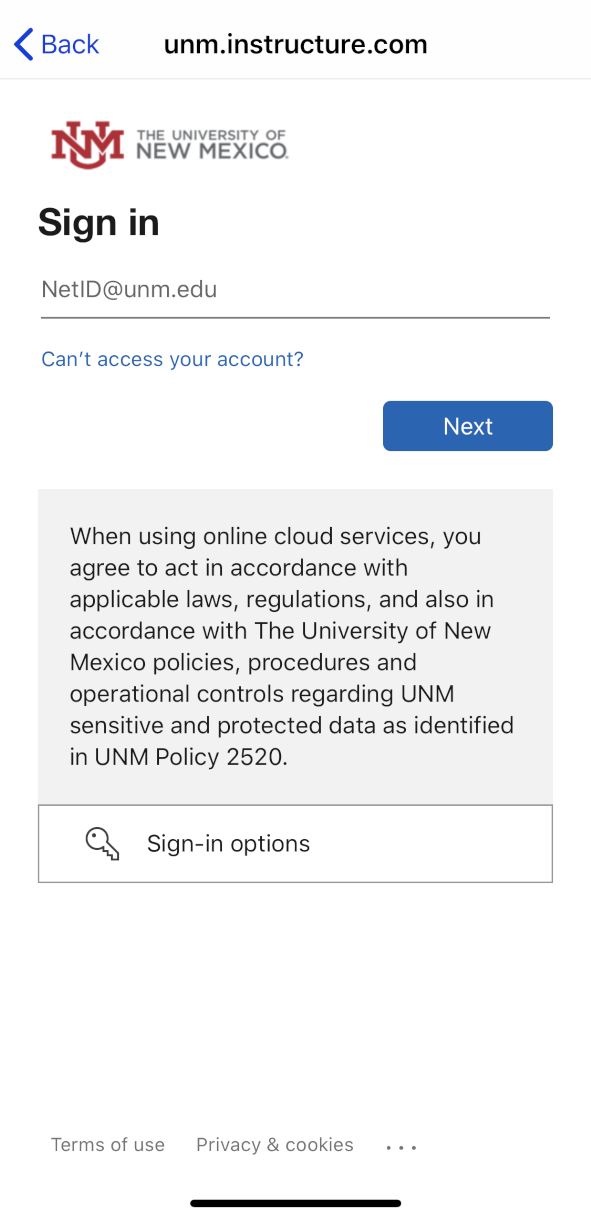The image depicts a detailed sign-in page for the University of New Mexico's online cloud services. 

- The interface resembles that of a mobile device, though no explicit indicators confirm this.
- At the top left, there is a "Back" button.
- The URL displayed is unm.instructure.com.
- The University of New Mexico logo appears prominently in red, featuring the letters "UNM."
- Below the logo, there's a prompt asking users to sign in using their NetID (netid@unm.edu).
- A blue hyperlink labeled "Can't access your account?" appears with a question mark.
- A "Next" button is visible to proceed with the sign-in process.
  
A message in a gray-shaded box informs users that by using these cloud services, they agree to abide by applicable laws, regulations, and the University of New Mexico’s policies, specifically UNM Policy 2520, which covers the handling of sensitive and protected data.

Additional features include:
- A "Sign-In Options" button bordered in gray.
- A key icon near the text "Sign-In Options."
- Links to "Terms of Use," "Privacy," and "Cookies" at the bottom, accompanied by an ellipsis (…). 

The page predominantly features blue, black, red, gray, and white colors with a primarily white background, except for the gray area containing the usage agreement text. Overall, the page is designed to authenticate UNM users while ensuring compliance with institutional data policies.